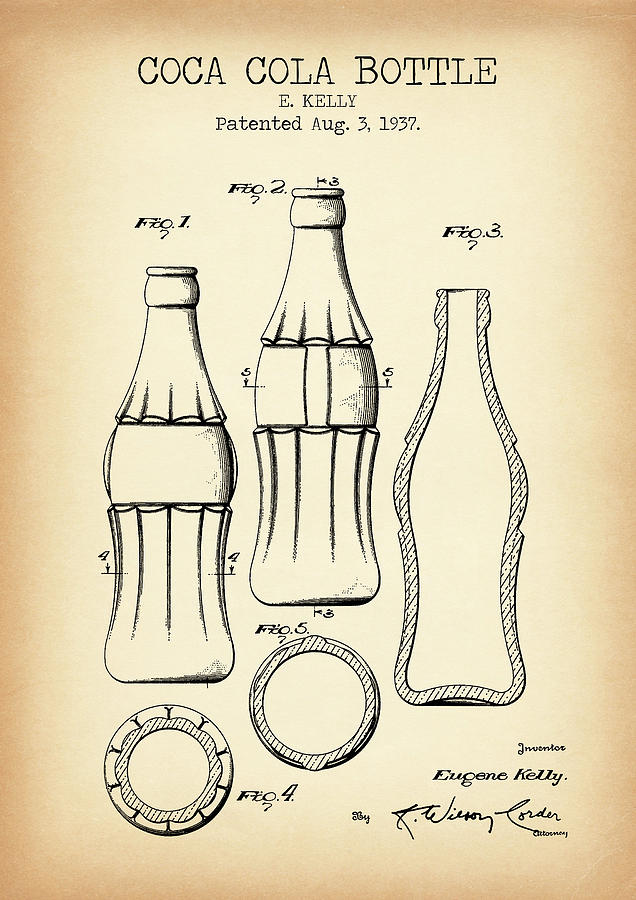The image is a detailed, weathered illustration of a Coca-Cola bottle patent dated August 3, 1937, by E. Kelly. The light brown paper features multiple black ink drawings, including three main profile views of the iconic hourglass-shaped bottle. The first two bottles are displayed fully while the third is a cross-sectional view that reveals the thickness of the glass, marked with black dotted lines along its edges. Above each bottle, there are small, unreadable black labels. At the top left, the text reads "Coca-Cola bottle E. Kelly patented August 3, 1937." 

Below the profile views, there are detailed illustrations of the bottle's bottom and cap, labeled as figures 1 through 5. Additional black text beneath these images states "Inventor: Eugene Kelly," and to the right, it features a signature, attributed to K. Wilson Lorder. The entire document serves as the original patent design for the Coca-Cola bottle, showcasing its distinctive and now familiar shape.